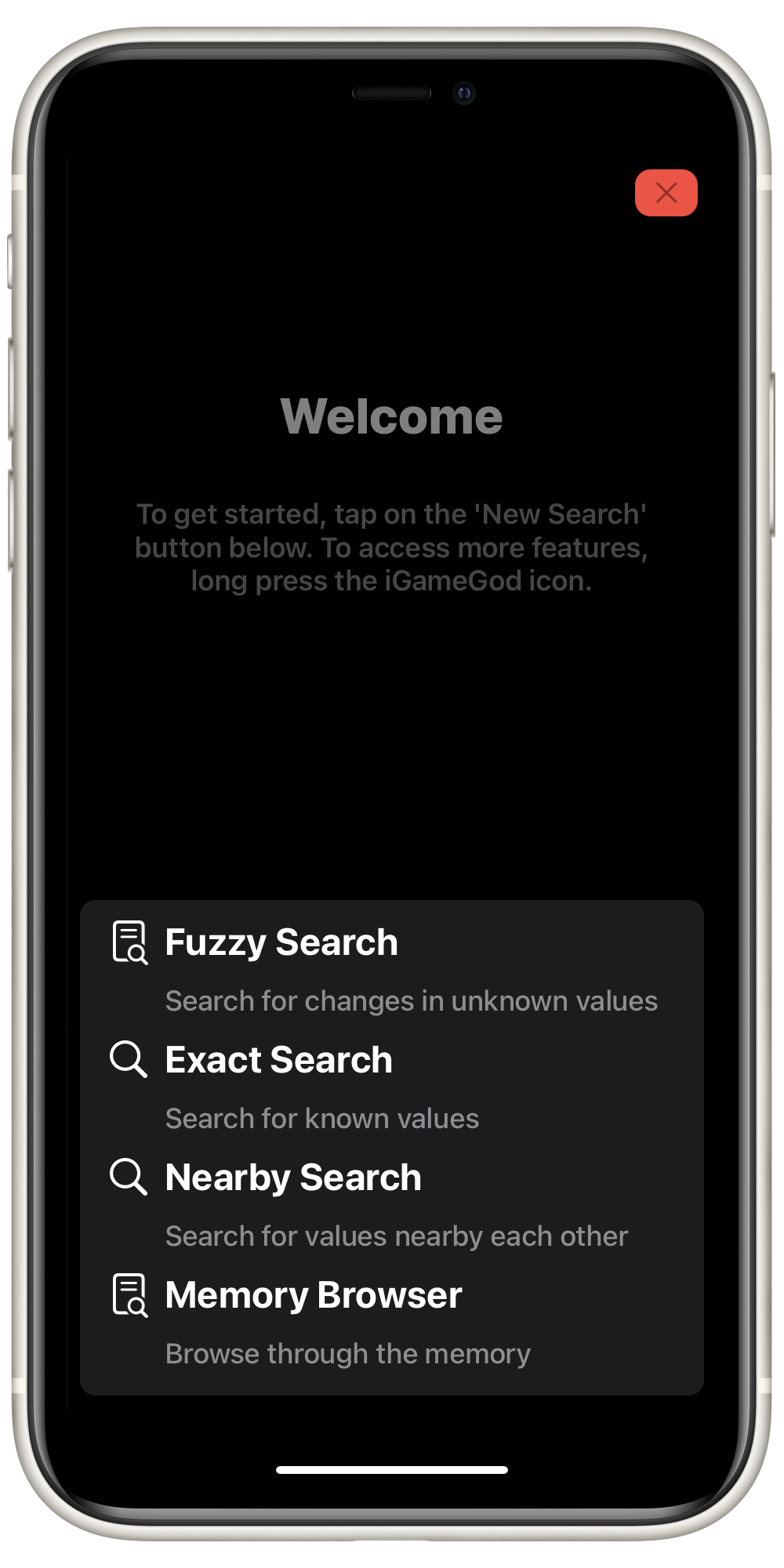The image features a black smartphone screen displaying a welcoming message. In the top right corner, there are two icons: a red 'X' and a square. The message instructs, "To get started, tap on the new search button below. To access more features, long press the iGame COD icon."

Beneath the introductory text, there are detailed descriptions of various search options:
1. **Fuzzy Search**: Accompanied by an icon, it allows you to search for changes in unknown values.
2. **Exact Search**: This option is for searching known values.
3. **Nearby Search**: It lets you search for values that are close to each other.
4. **Memory Browser**: This feature enables you to browse through the memory.

The search options and their descriptions are clearly displayed in white text against the black background, enhancing readability and visual contrast. The details are fairly explanatory, although not entirely comprehensive. It is not clear whether additional search options or browsers are available upon scrolling or if there is a next button to navigate to more features. The overall layout and crisp contrast make the instructions and options stand out prominently.